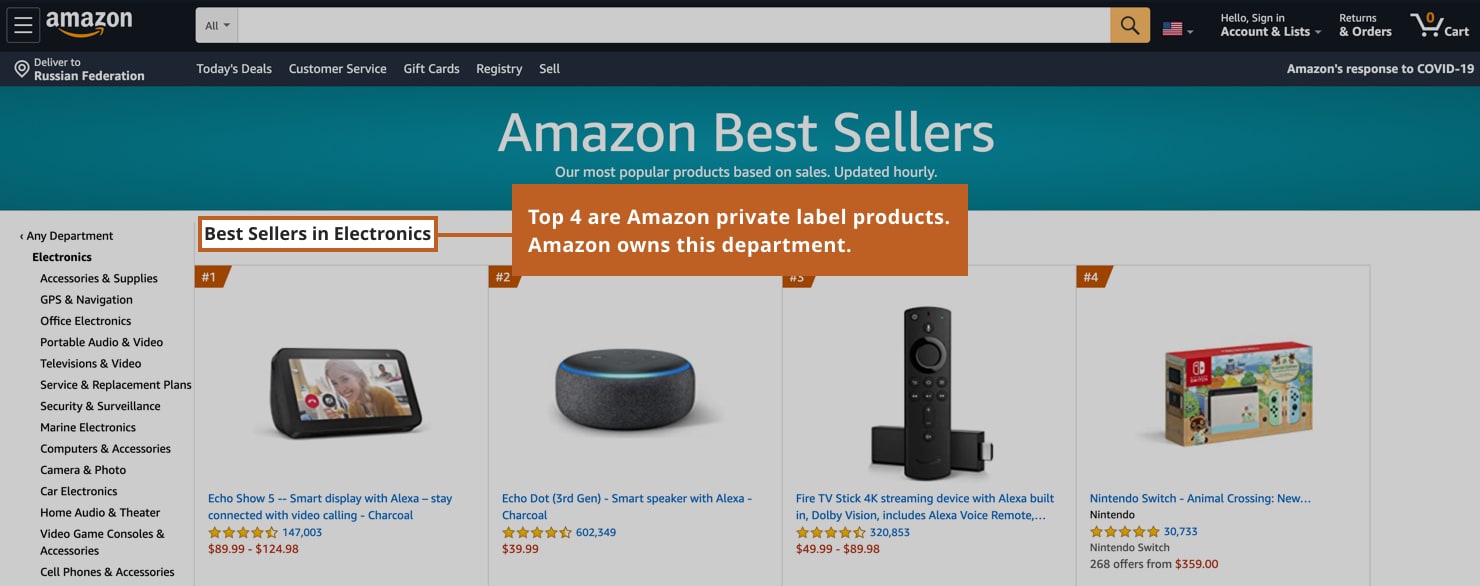The image displays a screenshot of a rectangular Amazon website page, elongated and stretched vertically. At the very top, a black navigation bar prominently features the Amazon logo on the upper left. To the right, options such as "Hello, Sign in," "Account & Lists," "Returns & Orders" are visible, along with a cart icon indicating it contains zero items.

Below this, a search bar allows users to find specific products. Directly underneath, a large blue banner reads "Amazon Bestsellers" in white text, followed by a subtitle stating, "Our most popular products based on sales. Updated hourly." This text is meant to draw attention to trending items.

An orange rectangle beneath the banner highlights that the "Top 4 are Amazon private label products," indicating Amazon's own line of goods. It points towards an orange-bordered section labeled "Bestsellers Electronics."

On the left side, the website lists various subcategories within the Electronics category, such as Accessories & Supplies, GPS & Navigation, Office Electronics, Portable Audio & Video, Television & Video, Service & Replacement Plans, Security & Surveillance, Marine Electronics, Computers & Accessories, Camera & Photo, Car Electronics, Home Audio & Theater, Video Game Consoles & Accessories, and Cell Phones & Accessories.

Finally, the right section of the site showcases four product images: various Amazon Echo devices and a Nintendo Switch, suggesting these items are top-selling or featured products in the category.